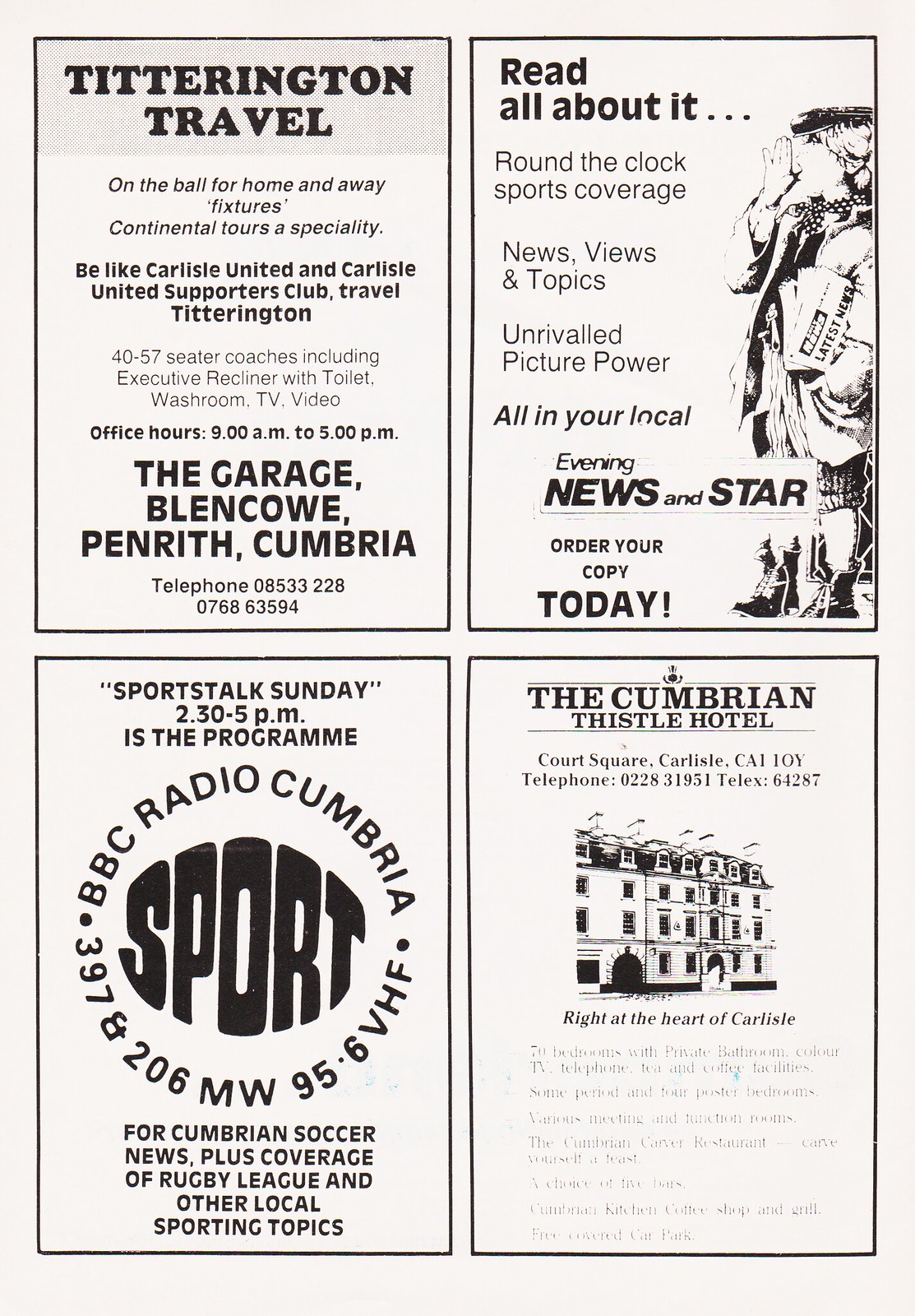The image features four vertically aligned tiles on a light gray background, each containing detailed information about different services. 

The top-left tile titled "Titterington Travel" in bold black text advertises a travel service that specializes in both home and away fixtures, as well as continental tours. The tagline reads, "On the Ball for Home and Away 'Fixtures'," and it encourages readers to "Be Like Carlisle United and Carlisle United Supporters Club, travel." It lists amenities for their 40-57 seat Cedar Coaches, including Executive Recliner with Toilet, Washroom, TV, and video, with office hours from 9 a.m. to 5 p.m.

The top-right tile promotes a news service with the headline "Read All About It," promising round-the-clock sports coverage and local news. It contains a sketched profile of a news carrier lady and emphasizes getting a copy of the local news, evening news, and star order.

The bottom-left tile advertises the "Cumbrian Thistle Hotel," featuring its telephone number and highlighting its prime location in the heart of Carlisle.

The bottom-right tile is dedicated to "Sports Talk Sunday," a BBC Radio program covering Cumbrian Soccer News, aired from 2:30 to 5:00 p.m. The entire image serves as a multi-faceted advertisement for travel, news, hotel services, and a radio sports program.